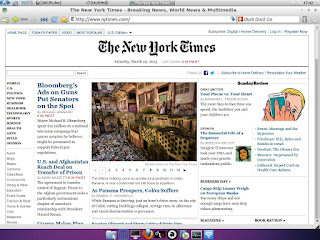In the image, someone is seen working on a computer. The screen displays an interface reminiscent of early 2000s bulky web browsers. Though the image becomes blurrier upon zooming in, several details are discernible.

At the top of the interface, various colors are visible: blue, black, green, and white. The black segments contain text that includes "New York Times," "breaking news," "world news," and "multimedia." There is a green arrow pointing to the left and a blue refresh arrow. Additionally, a white star with a green corner is seen, suggesting it might be an icon for bookmarking or favorites. The browser’s URL bar contains "www.nytimes.com" in black text. Another search box is present but the text within it is unreadable.

In the center, the screen prominently displays the New York Times logo. Below it, some black, gray, and red text is visible but remains too blurry to decipher precisely. On the left-hand side, blurred text in blue, black, and red reads snippets like "Bloomberg ads on guns, put senators on the spot" and mentions "U.S. and Afghanistan," although the details are indistinct.

The lower portion of the screen is less clear, showing an image that seems to depict rubble, though this is uncertain. Bottom-most elements of the screen include recognizable logos for a computer and the Firefox web browser.